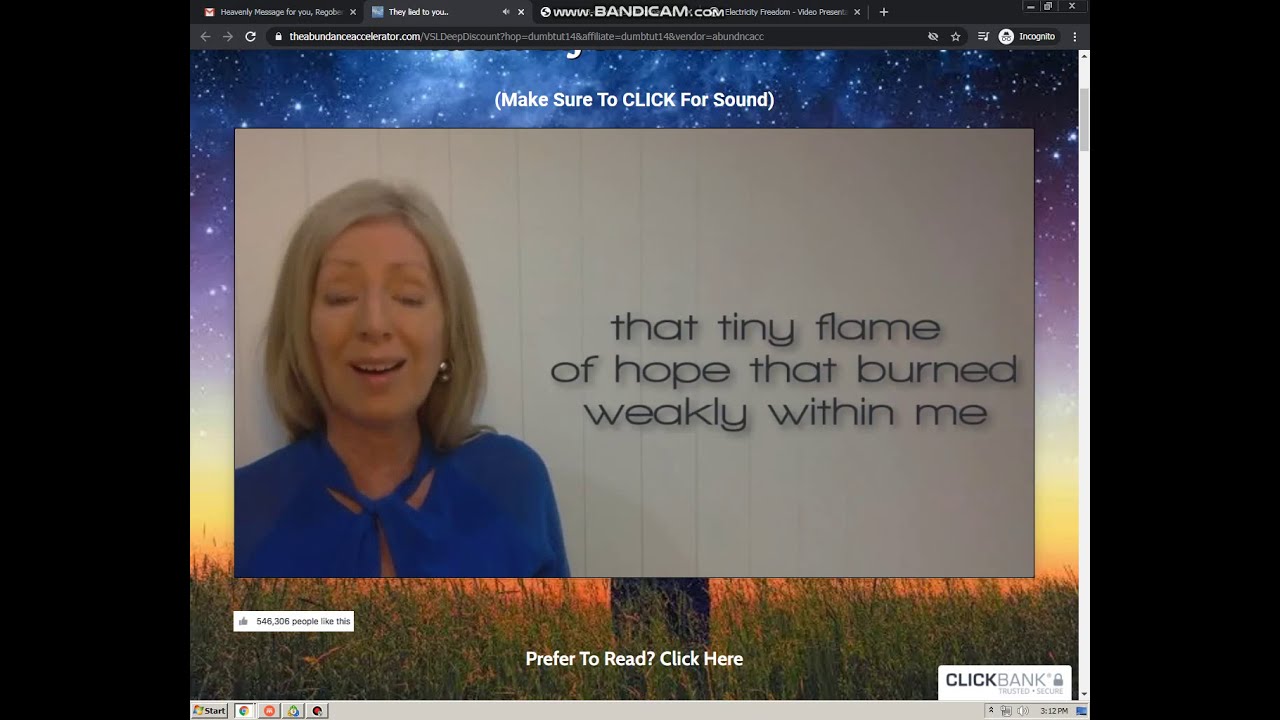The image is a screenshot of a webpage, displaying a visual mix of day and night elements in the background, with stars and a nighttime sky at the top transitioning to a lighter, daytime sky above a grass-covered ground. Dominating the left side of the image is a woman with closed eyes, dressed in a blue top, and standing against a white wooden board wall. To her right, there is text that poignantly reads, "That tiny flame of hope that burned weakly within me." Above, a heading instructs viewers to "Make sure to click for sound," suggesting the image is part of a clickable video. At the bottom, a call-to-action states, "Prefer to read? Click here." The screenshot, captured using Bandicam as indicated at the top, also reveals desktop elements like browser tabs, a Windows start button, and icons, highlighting that this is part of someone's computer screen. Additionally, there's a logo for ClickBank in the lower right corner.